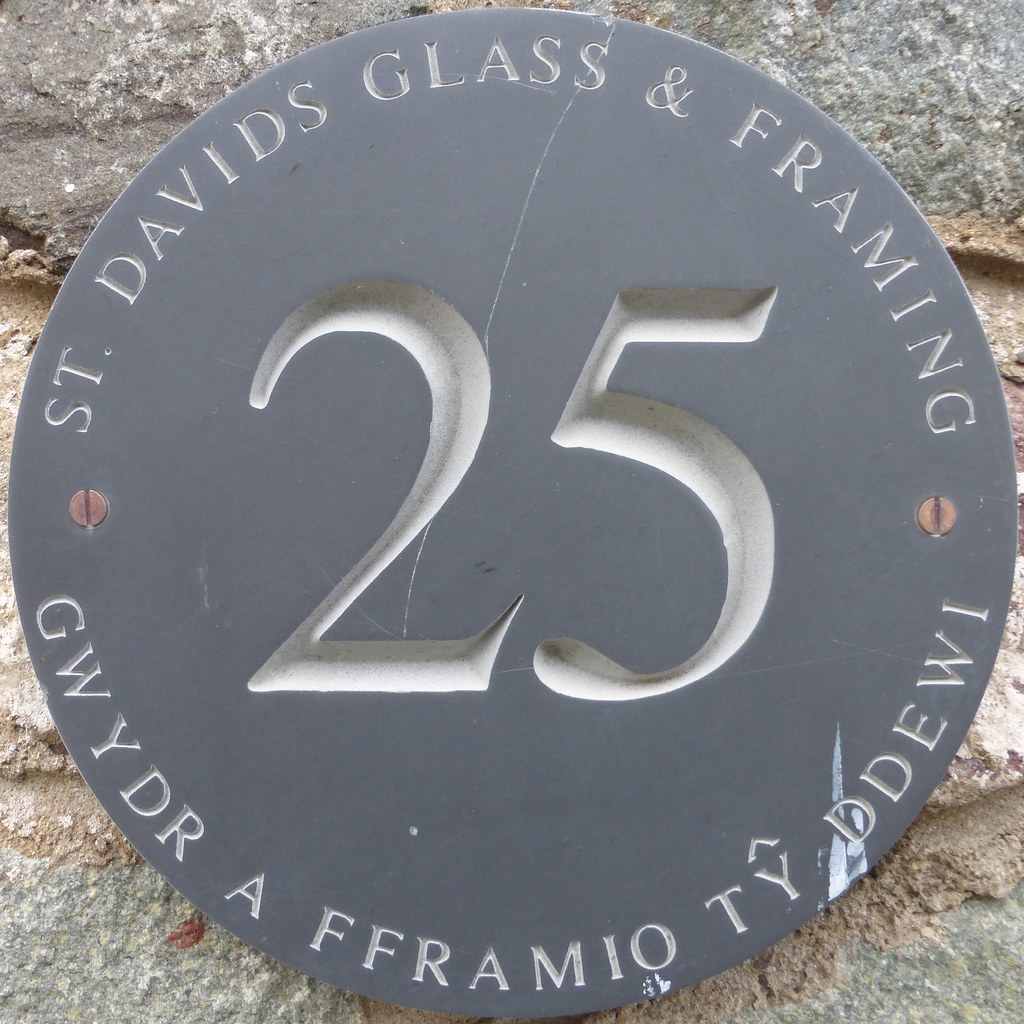This image features a round, gray metal plaque affixed to a stone wall, which varies in shades from medium gray to light brown. The plaque is secured with two screws, one on each side. Around the top perimeter in silver lettering, it reads "St. David's Glass and Framing," while the bottom perimeter displays the text "G-W-Y-D-R-A-F-F-R-A-M-I-O-T-Y-D-D-E-W-I," possibly in another language. Dominating the center of the plaque is the number "25" in large, light-colored font. The metal plaque shows signs of wear, with noticeable scratches, including a prominent one from the bottom of the "2" in "25" extending up to the "S" in "Glass," as well as additional markings on the lower right side. The setting, possibly commemorative, suggests it's celebrating 25 years of St. David's Glass and Framing.